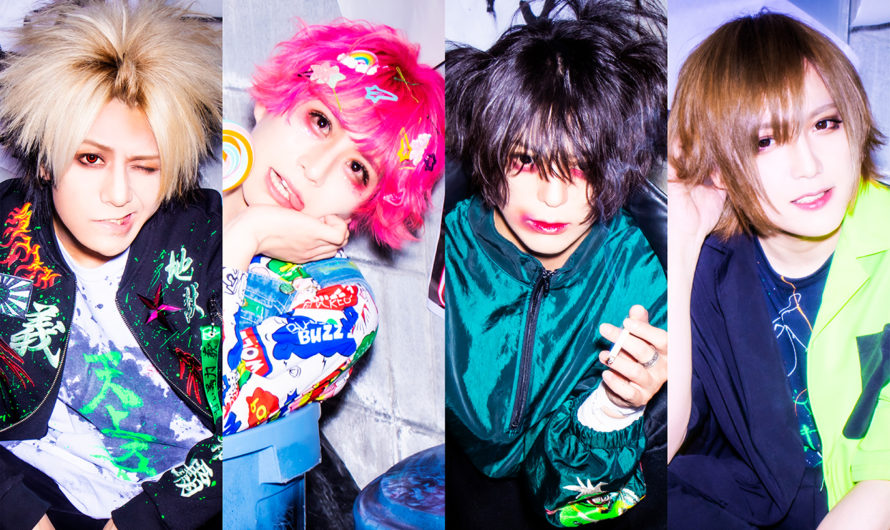The image is a composite of four vertical photos arranged in a horizontal row, showcasing different women with distinct facial expressions and vibrant outfits. On the far left is a woman with spiky blonde hair, described as looking like a mop on her head. She is wearing a dark blue jacket splattered with neon colors and possibly Chinese characters, along with a white t-shirt featuring splashes of green and blue. Her hands are barely visible at the bottom of the frame. To her right is another woman with short pink hair adorned with cute barrettes. She is making a silly face with her tongue sticking out and wearing a colorful, paint-splattered shirt bearing the word "Buzz." The next woman has short, messy brown hair, heavy smudged pink eye makeup, and a bright green jacket, holding a cigarette in her left hand and showing a smudged lipstick on her face. Finally, on the far right is a woman with short light brown hair, smiling with her teeth showing. She wears lipstick and a jacket that is dark blue on one side and green on the other. The carefully threaded-together photos create a vibrant collage of eccentric fashion and diverse expressions.